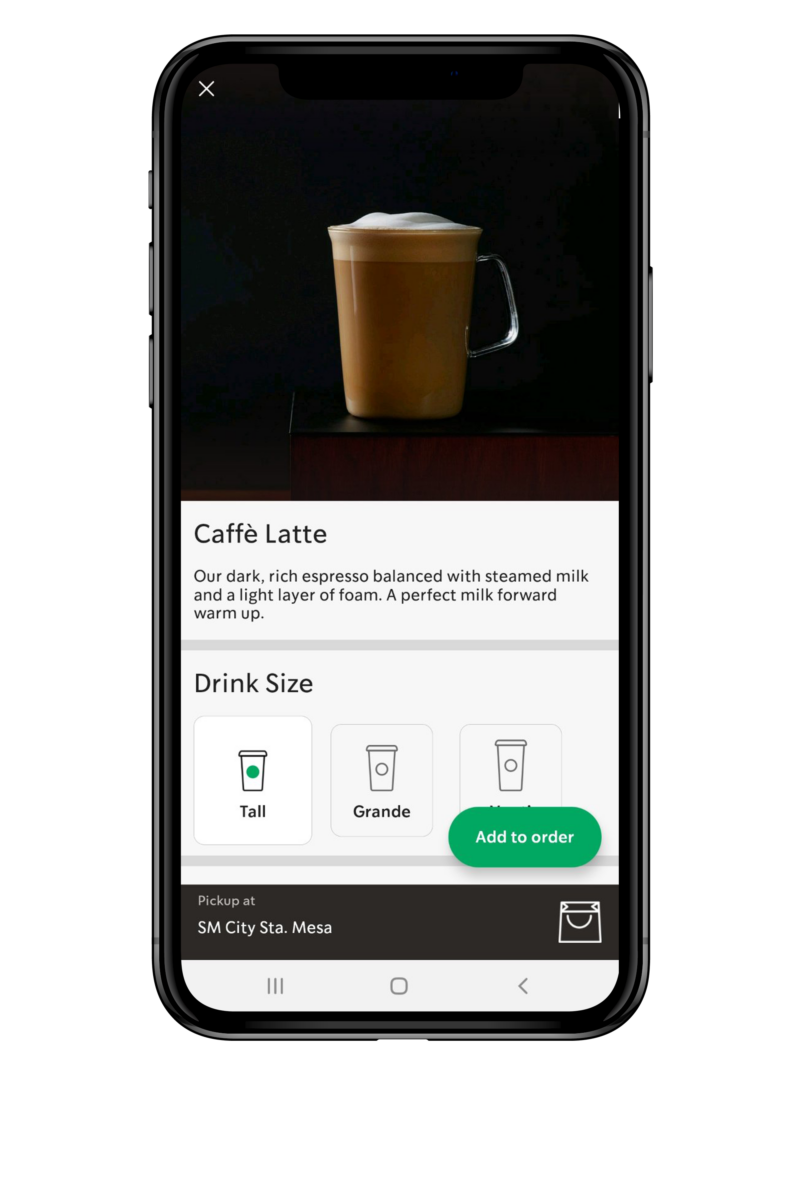The image showcases the front screen of an Apple iPhone displaying the Starbucks app. The app interface is currently on the page for ordering a café latte. The top half of the screen features a photo of a café latte, followed by a large black text that reads "Café Latte" on a white background. Directly below this, there is a short description of the drink in smaller black letters.

A thick gray bar divides the screen horizontally. Beneath this bar, the words "Drink Size" are prominently displayed in large black letters. Directly under "Drink Size," there are three cup icons representing the available sizes: Tall, Grande, and Venti. The green "Add to Order" button is situated in the bottom right corner, partially covering the Venti cup icon.

Below these elements, a black bar runs across the bottom of the screen displaying the words "Pick up at" followed by the address of the selected Starbucks location. On the right side of this bar, there is an icon of a shopping bag.